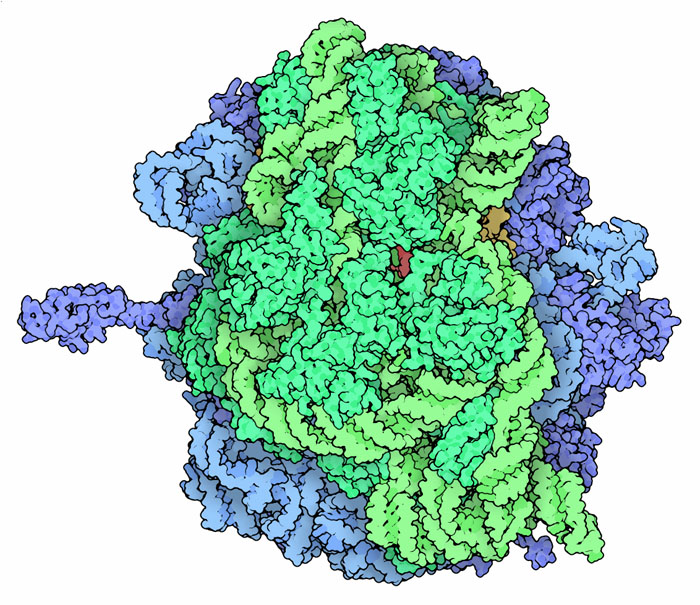The image appears to be a stylized, abstract piece of art on a clean, white background. It features a central, irregular mass of layered colors that resembles a porous, sponge-like or perhaps yarn-like structure. The outermost layer is a combination of periwinkle purple, violet blue, and light blue, which surround the entire mass in a jagged, circular motion. Moving inward, there are multiple shades of green—ranging from pea green and lime green to hunter green—creating a textured, crunchy appearance. Within this green area, particularly towards the center, there's a small, conspicuous section of burnt red or reddish burgundy, resembling a central node or focal point. Additionally, a tiny beige or brown segment can be found off to the side. The overall effect is akin to something squeezed out of a tube, layered in concentric circles, and tinged with a combination of cool and warm hues, evocative of various natural textures and forms.